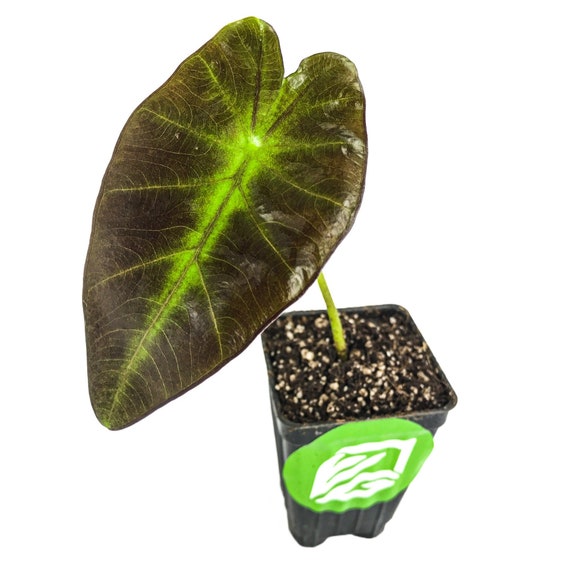This is an image of a single elephant ear plant viewed from above, set against a stark white background. The focal point is a large, heart-shaped leaf characterized by its dark green color and a striking, bright green central vein that branches out through the leaf's textured striations. The leaf extends to the left of the frame and exhibits a beak-like shape. The plant is potted in a small, black, square-shaped plastic pot adorned with a bright green label featuring a white leaf design. The pot contains dark soil interspersed with small white fertilizer beads. The stem, emerging centrally from the pot, accentuates the plant's lush and vibrant appearance despite the semi-blurry quality of the image.